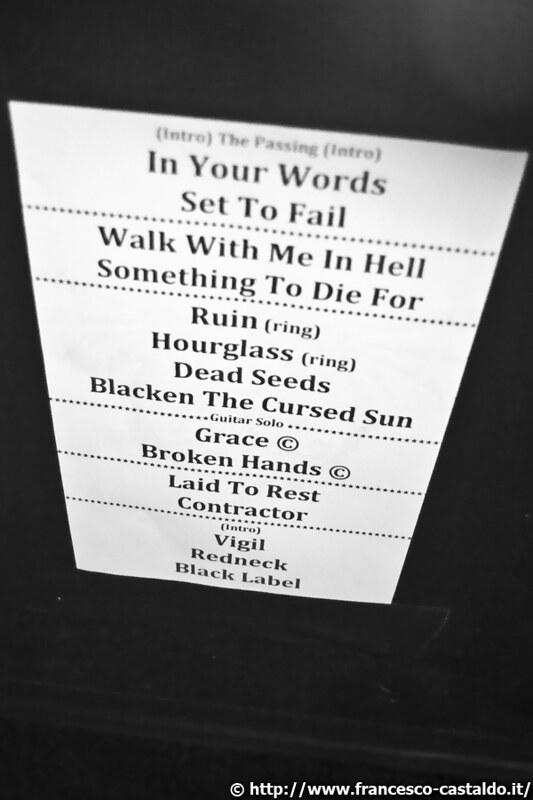The image is a black and white photograph of a setlist printed on a slim, vertical strip of white paper. The setlist text is rendered in black, centered, and segmented by horizontal dotted lines. The titles read from top to bottom as: "Intro, The Passing, Intro, In Your Words, Set to Fail," followed by a dotted line. Next, "Walk with Me in Hell, Something to Die For," followed by another dotted line. Continuing, there's "Ruin, Ring, Hourglass, Ring, Dead Seeds, Blacken the Cursed Sun," followed by a dotted line labeled "Guitar Solo." Then, "Grace ©, Broken Hands ©," followed by another dotted line. The sequence proceeds with "Laid to Rest, Contractor," then another dotted line. The final set reads: "Intro, Vigil, Redneck, Black Label."

The setlist is positioned at the center of the image against a predominantly black background, giving it a sharp contrast. At the bottom right of the image, there is a watermark in small white text that includes a copyright symbol and the URL "www.francesco.castaldo.it." The photo is taken from an angle that makes the bottom of the paper appear slimmer than the top. The texture of the paper suggests it is a standard sheet, potentially supported by a darker, indistinct surface at the bottom.